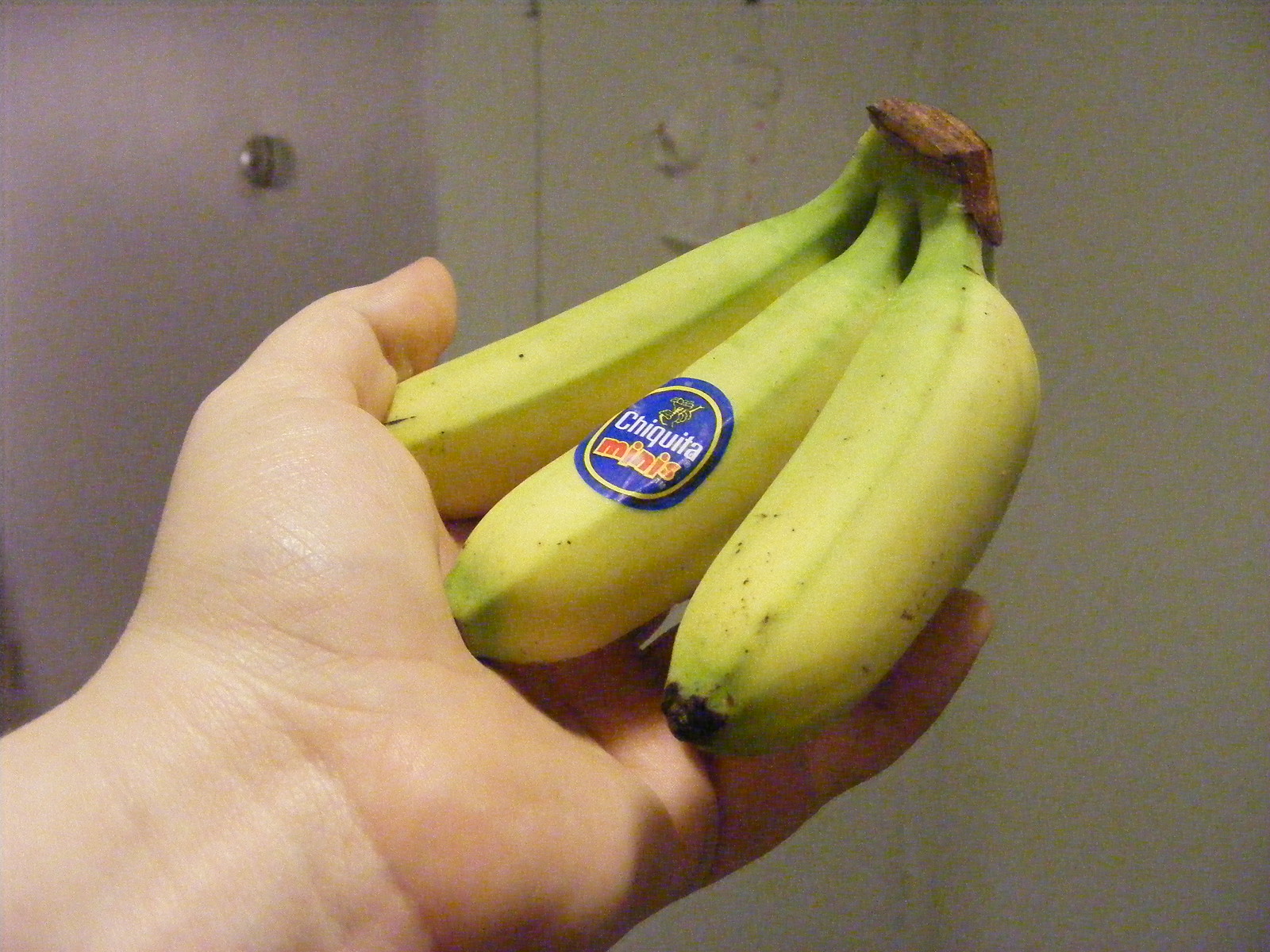This is a detailed color photograph taken up-close, featuring a person indoors. They are standing in front of pink and white-pink walls. Only the person's hand is visible, palm up, holding a bunch of bananas. The bananas are still attached by their stems, forming a small cluster of three.

A distinctive blue sticker with a yellow border, followed by another blue border, adorns one of the bananas. The sticker reads "Chiquita Minis" in white (for "Chiquita") and red (for "Minis") text. The bananas are predominantly yellow with shades of green towards both the ends – transitioning from green at the stem, through yellow, and back to green at the bottom.

Among the three bananas, one appears slightly more ripe with a few brown spots and a browning bottom, unlike the greener ends of its counterparts.